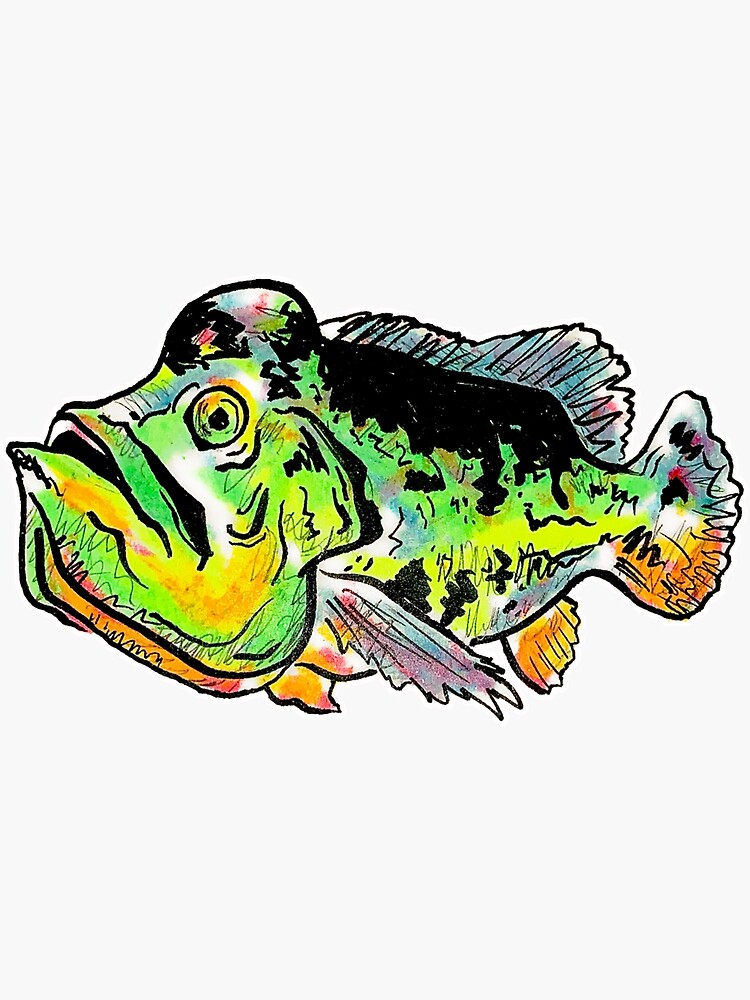The image showcases an illustrated drawing of a fish against a completely white background. The fish, potentially a largemouth bass given its mouth size and shape, is depicted with a bright, tie-dye blend of psychedelic colors. The head of the fish features a vivid mix of pink, red, green, light blue, white, and orange hues. Its underside is predominantly red with orange beneath the mouth; the chin appears distinctly white. The fish's dorsal fins and tail fin are adorned with intricate scribbles, adding a cartoony effect. The fish's body transitions through black, green, yellow, and blue, accented by a dark black streak along its back which almost gives an impression of hair or foliage. The back fins are blue and pink, while the bottom fins are pink and blue. The tail fins showcase a striking combination of red, yellow, blue, purple, white, and black. The fish's eye, seemingly looking out of the image, and the slight gap of its open mouth complete the detailed, animated appearance of this colorful aquatic illustration.